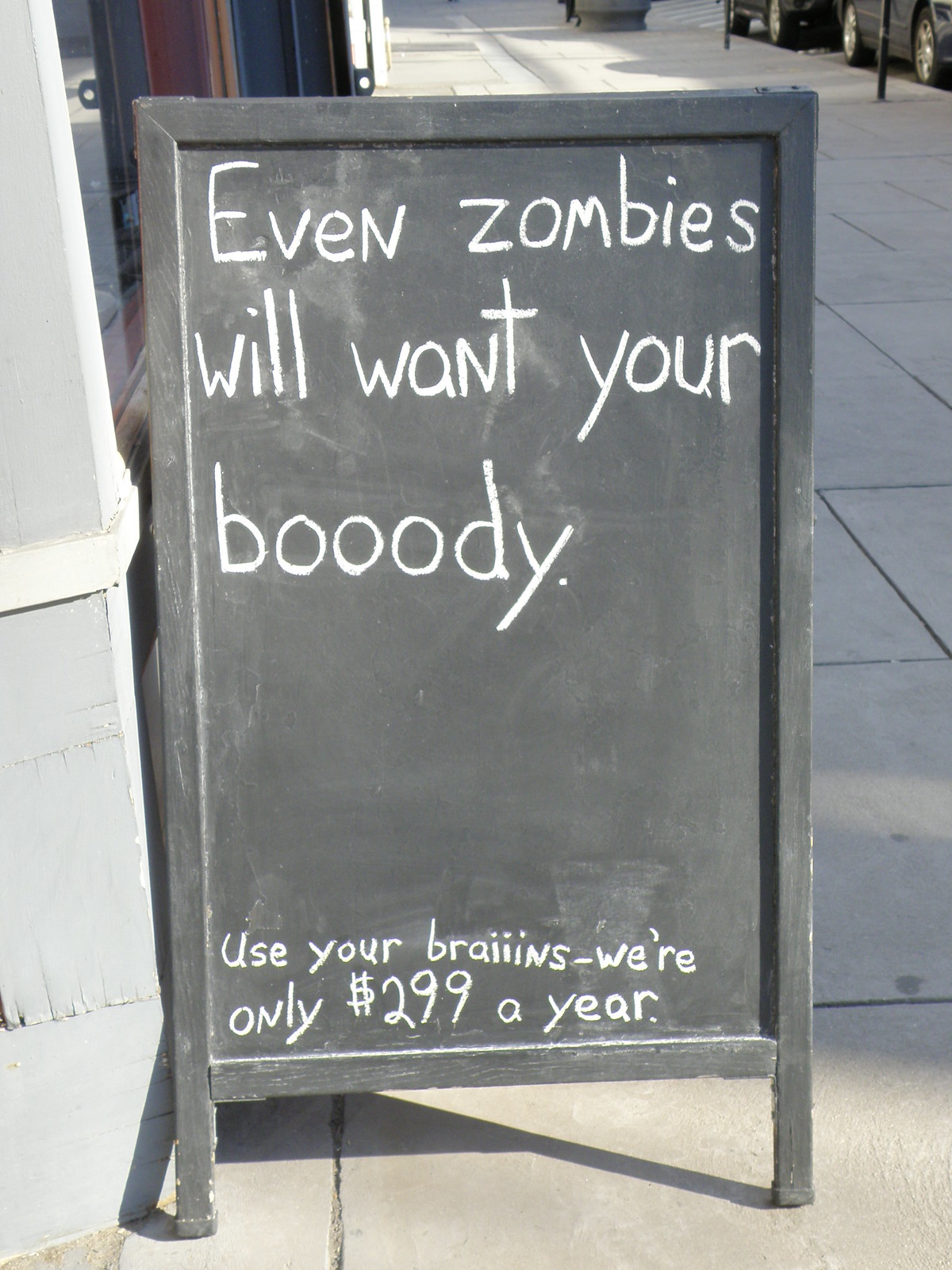This image depicts a black chalkboard-styled sign with a black wooden frame, standing on a neatly paved gray sidewalk outside of a business. Written in white chalk are the phrases: "Even zombies will want your bOOody" and "Use your braiiins" followed by "We're only $299 a year." The blackboard is leaning against a gray building wall, contributing to the overall gray theme of the surroundings. In the background, a few parked car wheels are visible, adding a subtle hint of an urban outdoor setting. The area appears devoid of any people, focusing solely on the cleverly written sign attempting to attract customers to the business.